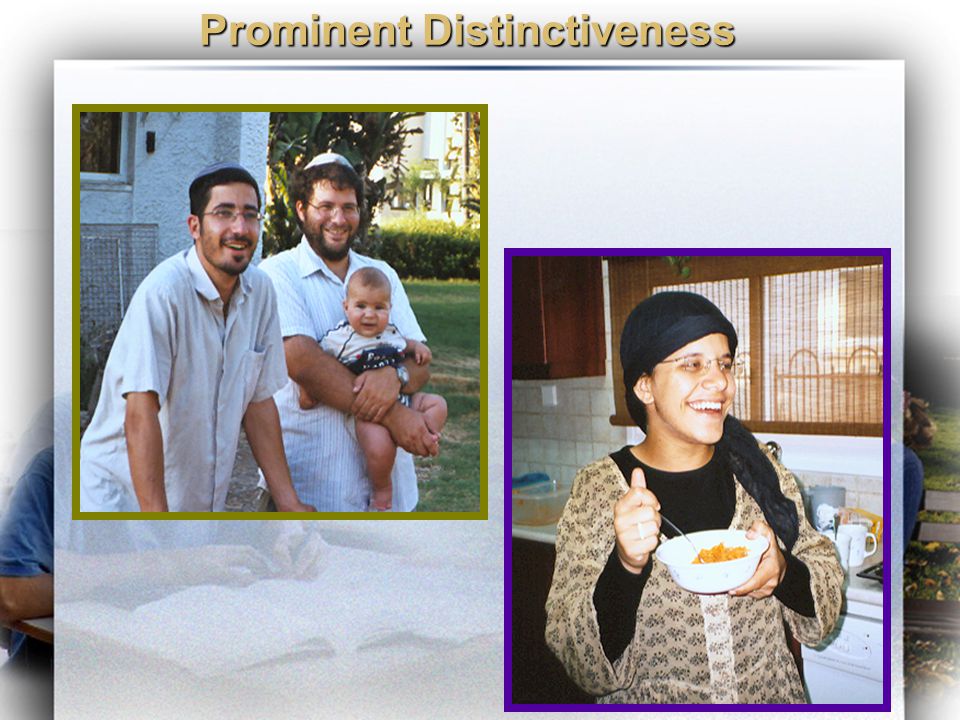This image, titled "Prominent Distinctiveness" in gold letters, features a photo montage with a white background. The montage is composed of two main pictures outlined in different colors. 

The first picture, located on the left, depicts two men with glasses and beards. The man on the left has black hair, while the man on the right, who is holding an infant, has brown hair and a yarmulke. Both men and the baby are dressed in white. The background reveals a blend of green grassy areas, white buildings, and bushes, giving an outdoor setting feel.

To the right, diagonally, is the second picture outlined in purple. This picture shows a woman smiling as she eats a bowl of cereal. She is wearing a black shawl on her head, a black shirt, and a tan over shirt with a pattern. The background appears to be a kitchen, with details including white-tiled walls, brown cabinets, a silver-colored bench, windows with blinds, and various kitchen utilities and utensils.

All these elements come together to create a visual contrast between the two distinct scenes, emphasizing the theme of "Prominent Distinctiveness."